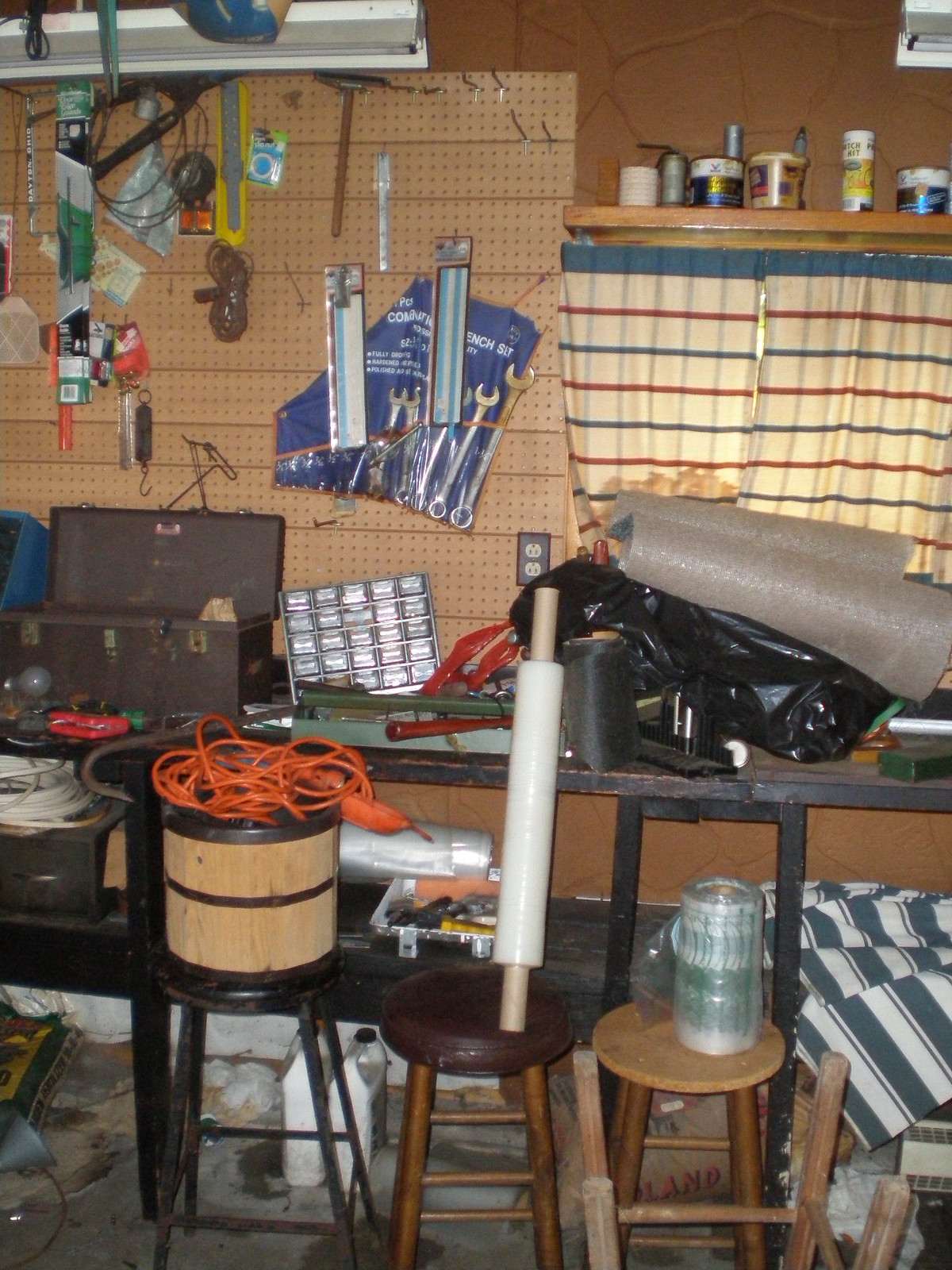This photograph captures a detailed view of a well-organized workshop. The back wall is constructed from a rustic brown stone, providing a sturdy backdrop for the workspace. Dominating the wall are several pegboards, each filled with evenly spaced holes and adorned with metal pegs. Various packages and tools hang neatly from these pegs, showcasing the efficient use of space from the left side towards the center and extending further to the right.

To the right side, a high wooden shelf catches the eye. Draped from this shelf is a striped cloth in black, dark blue, red, and cream tones. Atop the shelf, several cans containing different types of products are meticulously arranged. Just beneath this arrangement, a long workbench spans the width of the photograph, providing ample workspace for various tasks.

On the left side of the bench, a metal tool case is prominently placed, surrounded by a multitude of items essential for handiwork. Below the workbench, an additional shelf houses an assortment of items including extension cords, wiring, plastic wrap, and possibly a tarp. Adding to the workshop's functionality, a few small round wooden tables with slender legs are positioned beneath the bench, ready for use whenever needed. The overall scene presents a lively and practical environment, rich with tools and materials ready for any project.